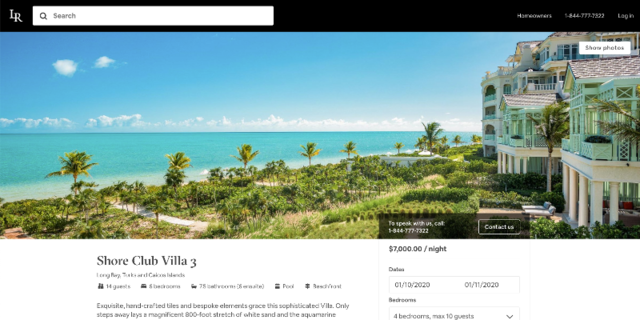The webpage in question appears to be from a resort or hotel vacation booking website, with a logo featuring the initials "LR" in the upper left corner, set against a black background. Despite the slightly blurred web address and site name, a phone number and login option are visible at the top.

The main feature on the page is the "Shore Club Villa 3," accompanied by an image of an elegant beachfront villa, showcasing pristine blue waters, lush island-style foliage, and manicured grass. The villa itself is painted in a mix of white and pastel green, featuring stately pillars at its base, indicating a large and luxurious property.

The villa is advertised at $7,000 per night. Below the image, there is some text highlighting the villa's unique aspects, such as exquisite handcrafted tiles and bespoke grace, although part of the description is cut off. We learn that the villa is merely steps away from an 800-foot stretch of white sand and aquamarine waters.

To the side, there is a contact number, 1-844-377-732, along with a "Contact Us" button. Potential guests can also see availability dates listed as January 10, 2020, to January 11, 2020. The villa accommodates up to 10 guests across its four bedrooms. The sky in the background of the image is notably bright and picturesque, adding to the overall allure of the destination.